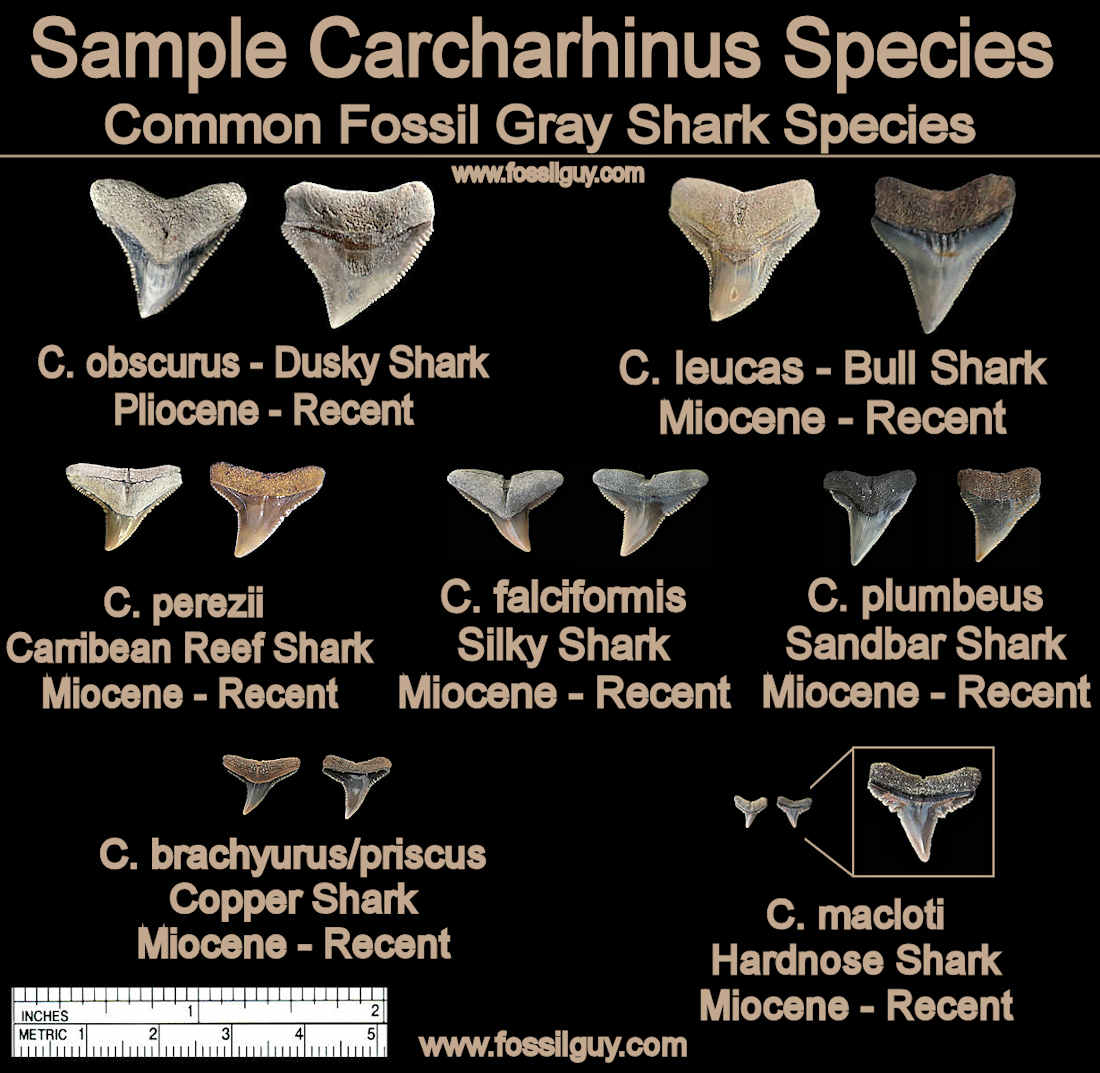The image features a detailed computer display of various shark teeth, showcasing specimen from common fossil gray shark species, specifically within the genus Carcharhinus, a prominent family of sharks. The background is black, with all the lettering highlighted in pink, including the title "Sample Carcharhinus Species" and the website "www.fossilguide.com." Presented within the display are photographs of 15 different types of shark teeth, meticulously labeled with their respective species and geological epochs.

Prominently displayed at the upper left is the tooth of a Carcharhinus obscurus, known as the dusky shark, which has serrated, wide, sharp-pointed teeth dating back to the Pliocene Epoch. Adjacent to it is the Carcharhinus leucas, or bull shark, possessing narrower, sharply pointed teeth from the Miocene Epoch. The Caribbean reef shark, Carcharhinus perezi, follows in the middle, represented by even narrower teeth with serrations along the edges.

Further along, we observe the Carcharhinus falciformis, commonly known as the silky shark, which features very narrow, shorter teeth, and the Carcharhinus plumbeus, or sandbar shark, with slightly longer but similarly shaped teeth. The copper shark, Carcharhinus brachyurus/priscus, showcases extremely narrow teeth, while the hardnose shark, Carcharhinus macloti, presents narrow but relatively long teeth at the bottom of the display.

A ruler is included at the bottom of the image for scale reference, enhancing the scientific accuracy and providing context to the various tooth sizes. All teeth in this educational graphic span from the Miocene to recent geological periods, offering a comprehensive overview of these predatory species' dental evolution.